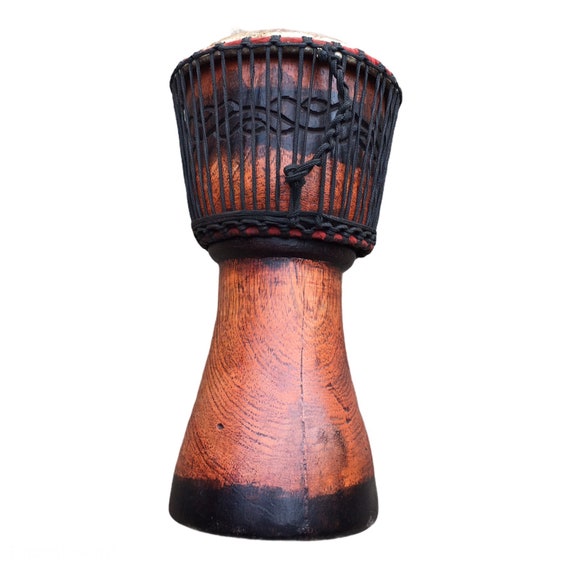This image features a traditional, handcrafted wooden drum, distinctly different from typical band drums and richly reflecting its native cultural roots. The drum is short, somewhat resembling an hourglass in shape. A closer look reveals its natural wooden brown hue, accentuated by black and reddish tints. The base of the drum is stained black, and its central body showcases the wood's natural red tones and grain. Along the top section, a black band with intricate swirling carvings encircles it, adding a decorative touch. The drum's upper surface is covered with a white material trimmed with red. Braided black rope, vertically arranged, adorns the top portion, creating a handle-like feature, while a piece of this cord dangles from the side. The overall craftsmanship, including the carved patterns and corded elements, highlights the drum's traditional design and handmade quality.